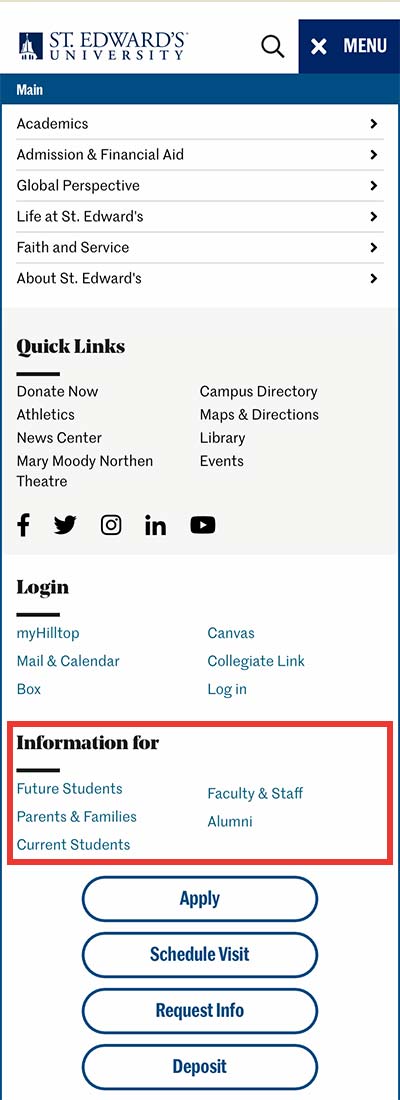The image is a detailed screenshot from a smartphone or tablet, depicting an interactive webpage for Saint Edward's University. 

At the top of the screen, a dark blue square icon with a white building and a flag set against a blue background is visible. Next to the icon, the text "ISTE for Saint Edward's University" appears in dark blue letters. To the right, there's a black magnifying glass icon for search functionality. Adjacent to it, a dark blue rectangle with a bold white "X" and "MENU" in white bold text is situated. Below it, another smaller dark blue rectangle displays "MAIN" in bold white text on the left side.

The main section showcases a dropdown menu featuring various selections, each accompanied by a black right-pointing arrow and formatted in bold black text. The options listed are:
- Academics
- Mission and Financial Aid
- Global Perspective
- Life at Saint Edward's
- Faith and Service
- About Saint Edward's

Underneath this dropdown, a light gray rectangle contains "QUICKLINKS" in bold black text with an underline. Below this title, several quick access links are arranged in alternating left and right alignment:
- Donate Now
- Campus Directory
- Athletics
- Maps and Directions
- News Center
- Library
- Moody Northern
- Events
- Theater

Beneath the quick links, several social media icons in bold black are listed, including:
- Facebook (lowercase "f")
- X (formerly known as Twitter) with a tweeting bird icon
- Instagram (rounded square with two circles)
- LinkedIn (lowercase "in")
- YouTube (rounded square with an upturned white triangle)

Following this are login options in bold black text with an underline, and hyperlinked blue text with various services. The options on the left side are "My Hilltop," "Canvas," "Mail and Calendar," "Collegiate Link," and on the right side "Box" and "Log in."

A red rectangle outlines a specific area the screenshot's taker wishes to highlight. The area marked by the rectangle contains "Information For" in bold black text followed by a small black line. Beneath this, more hyperlinked blue text is provided, listed in a left-to-right arrangement:
- Future Students
- Faculty and Staff
- Parents and Families
- Alumni
- Current Students

At the bottom, there are multiple clickable buttons in dark blue with dark blue borders, offering:
- Apply
- Schedule a Visit
- Request Info
- Deposit